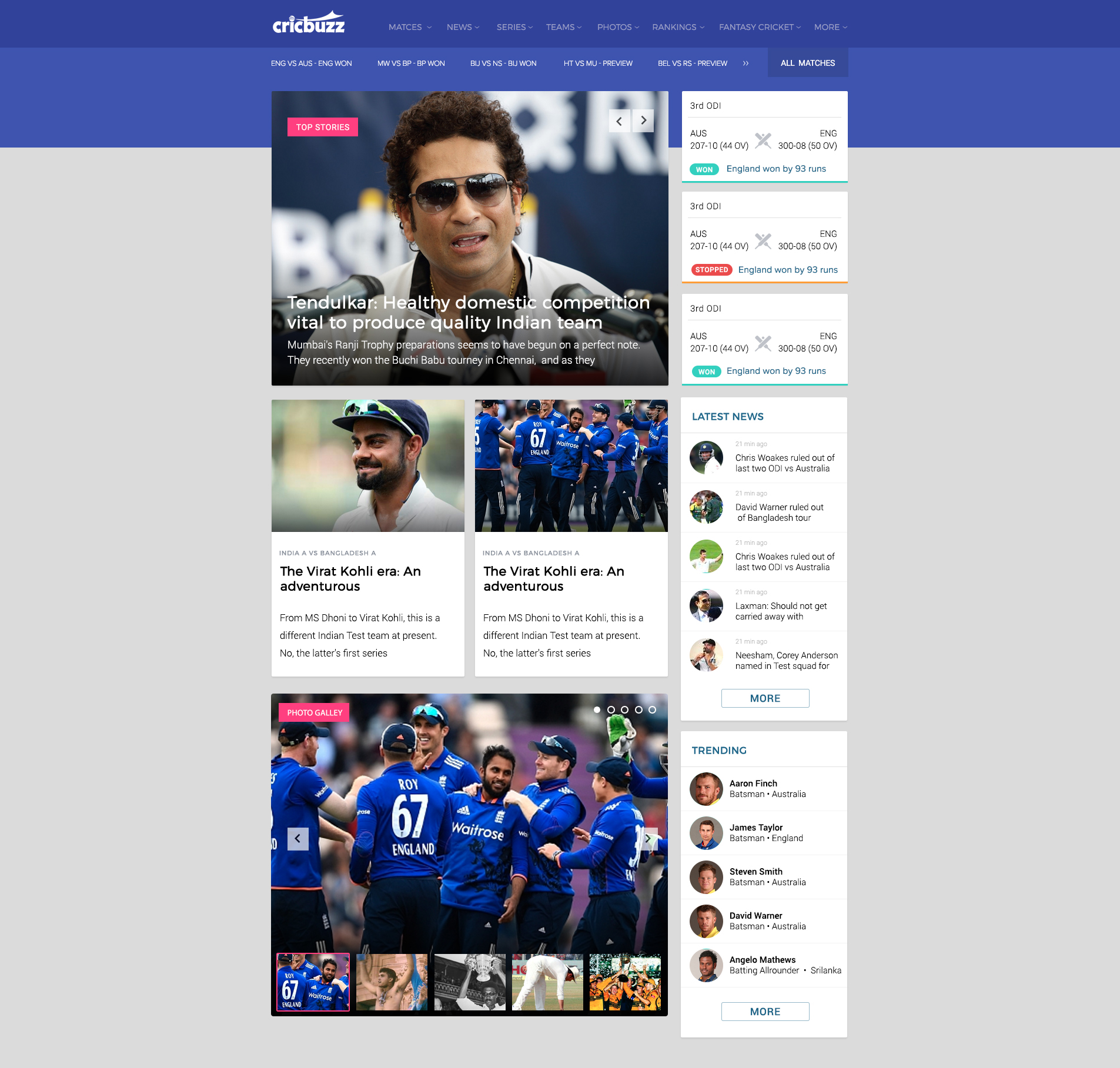This image is a screenshot from a website featuring a predominantly blue header that gradually transitions from a darker to a lighter shade. At the very top of the blue background, the website's name, "Cricbuzz," is prominently displayed. Adjacent to the site's name are navigation options such as News, Game, Photos, and more. Below the lighter blue section, text in white, though blurry, appears to provide additional information.

The main content area of the website has a gray background. The top article features a large image of a man wearing sunglasses speaking to several microphones. This article appears to discuss producing a quality Indian team. Below this, additional articles follow, all seemingly related to sports topics. On the right side of the page, there are clickable sections labeled "Latest News" and "Trending," offering users quick access to the most current and popular content.